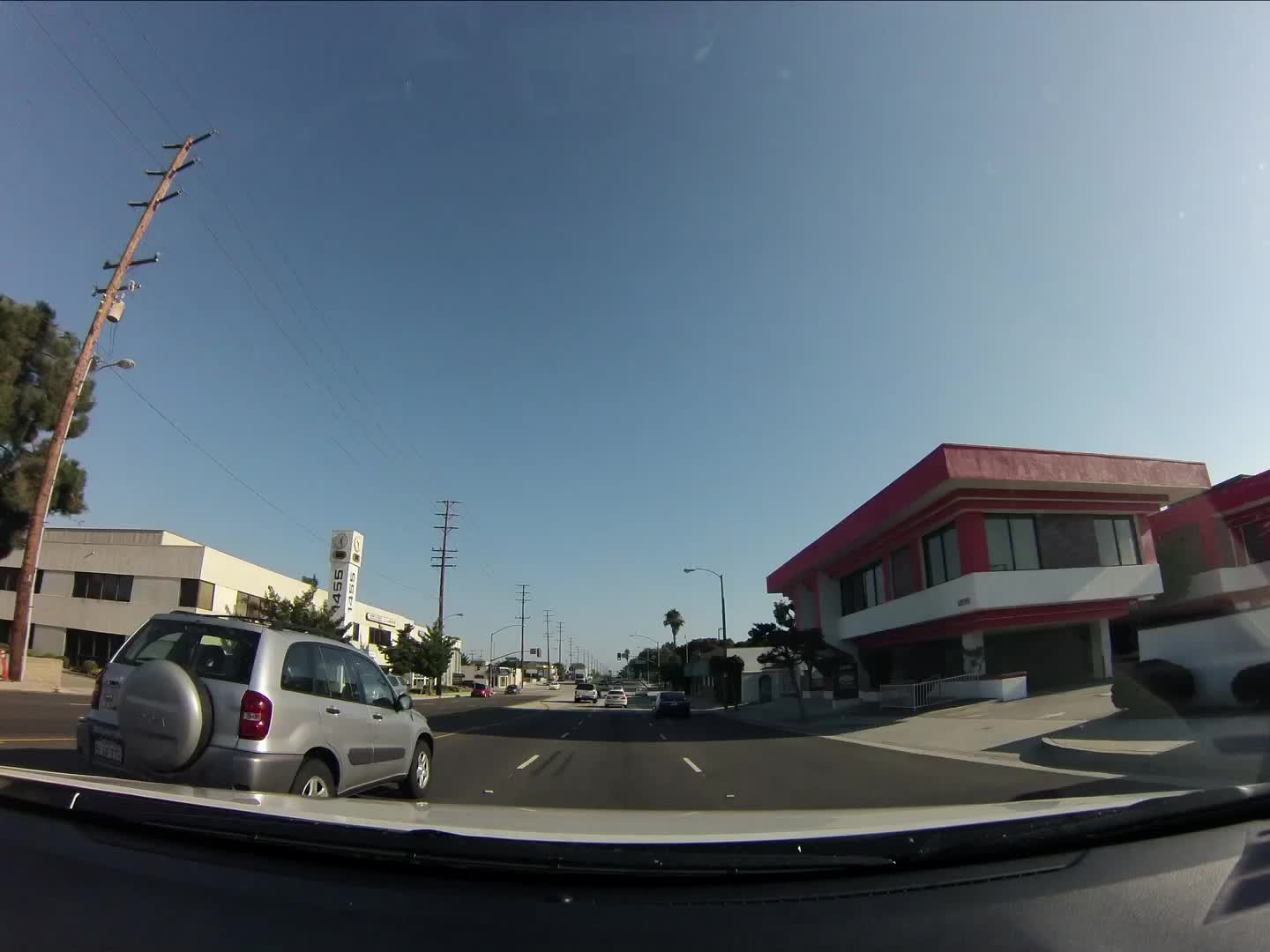This is a daytime photograph taken from inside a northbound vehicle situated in the middle lane of a three-lane road. The hood of the car, which is white, can be seen prominently in the foreground. Ahead and slightly to the left, there's a gray vehicle. To the right of the car, a red building with accompanying structures is visible. A power line runs along the left side of the image, paralleling the road. Multiple other cars can be seen both in front of the vehicle and on the opposite side of traffic. The lighting indicates that the sun is in the upper right-hand corner of the frame, casting brighter shades and creating a white hue in that area.